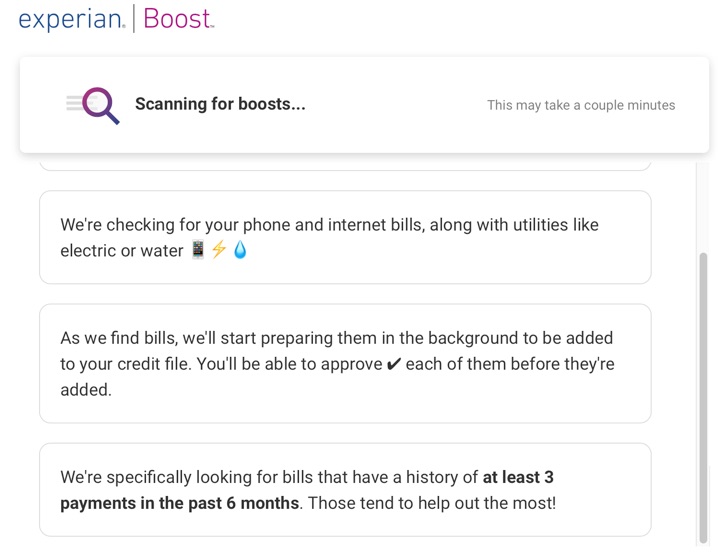This screenshot captures the interface of a website called Experian, prominently displaying the feature "Boost" at the top left corner. The concentrated activity on the page shows the system engaging in a scanning process, indicated by the text "Scanning for Boost..." alongside an animated magnifying glass icon to its left, suggesting a search operation is underway. Beneath this, a message informs the user that "This may take a couple of minutes," implying that an analysis or loading process is occurring.

Following this, the interface lists several key updates linked to the scanning action:
1. A notification states, "We're checking for your phone and internet bills along with utilities like electric or water," accompanied by emojis representing a phone, an electrical plug, and a water drop.
2. An explanation reads, "As we find bills, we'll start preparing them in the background to be added to your credit file. You'll be able to approve ✅ each of them before they're added," with a checkmark emoji highlighting the approval process.
3. The final message details, "We're specifically looking for bills that have a history of at least three payments in the last six months. Those tend to help out the most," underlining the criteria for bill selection focused on enhancing the user's credit file.